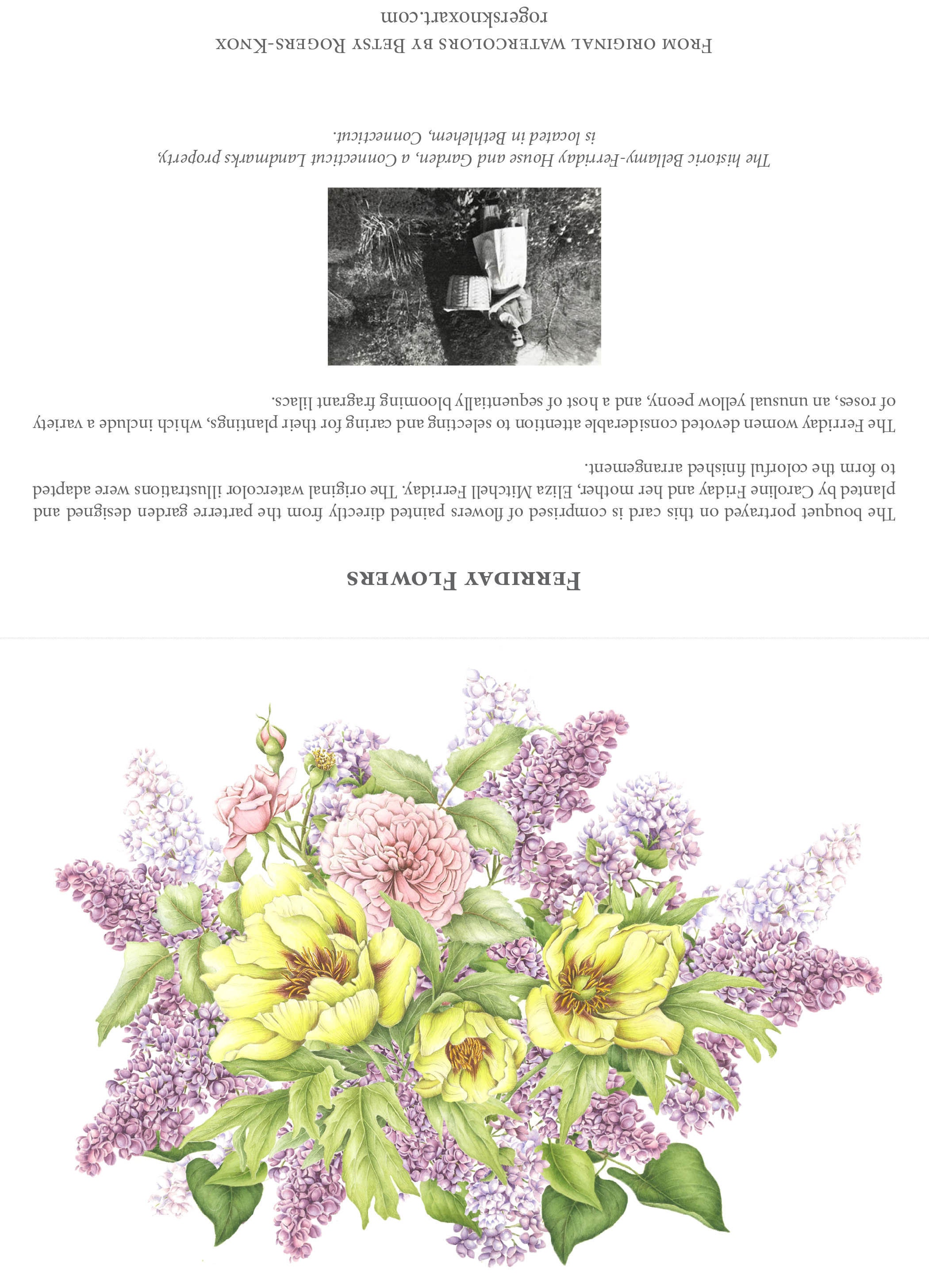This is an upside-down scan of a detailed greeting card featuring vibrant floral artwork and descriptive text. The bottom half showcases a large, colorful bouquet with a variety of flowers: central yellow flowers with brown seeds, surrounded by green leaves, tiny purple flowers, and a prominent pink flower. The edges of the bouquet display lilacs in purple, wild roses in soft yellow and white, and a pale purple chrysanthemum. Above the bouquet, a subtle gray line separates it from upside-down text, beginning with the title "Faraday Flowers." This is followed by two paragraphs of left-aligned text describing the imagery. A small, black and white, horizontally aligned, rectangular photo shows a woman holding a basket, standing next to buckets and trees with lush greenery in the background. Italic text follows beneath her image, concluding with the phrase "From Original Watercolors by Betsy Rogers Knox" along with a website, rogersknoxart.com.